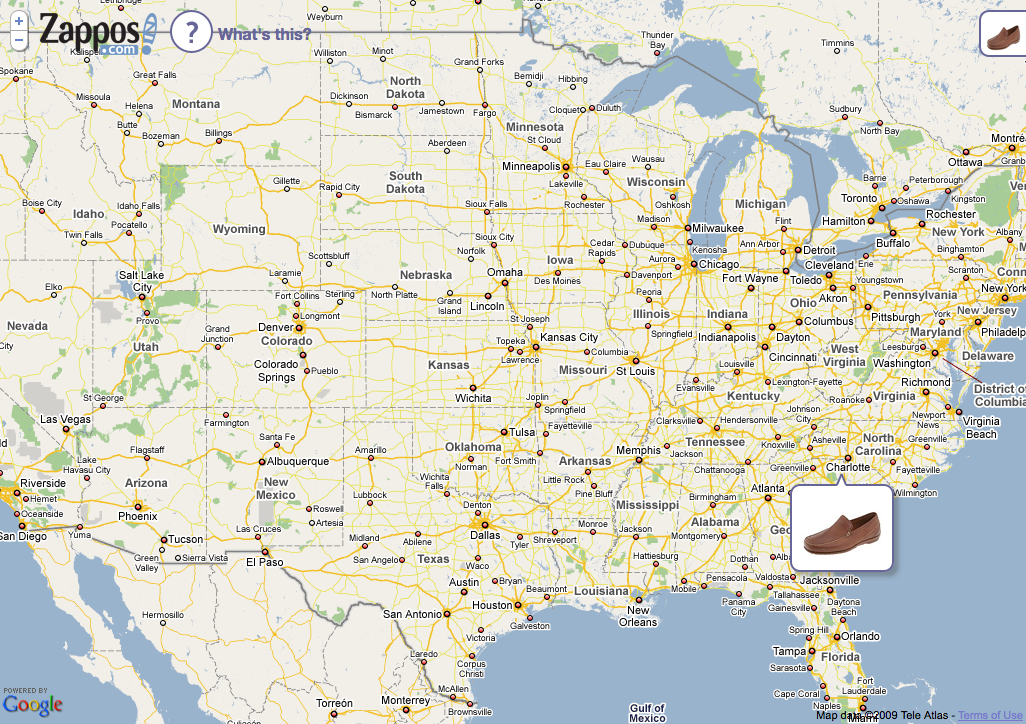This image shows a highly detailed, color map of the United States, clearly presented by Google, featuring an extensive range of cities, including both major and smaller ones like Pine Bluff, Arkansas, and Little Rock. Prominently, the map includes a shipment locator for Zappos. 

In the North Carolina area, there is a brown loafer shoe icon pointing specifically at Charlotte, North Carolina. A similar icon appears in the top right-hand corner, though it is partially cut off. The map offers detailed geographical features, showcasing rivers, the Great Lakes, and oceans in blue, as well as green areas representing various terrains. You can also see the southern part of Canada, particularly southern Ontario, and northern Mexico, though half of California is cut off from view.

Additional elements include a zoom in and zoom out button, the word "Zappos" next to it, and a circle with a question mark inside, labeled "what's this?" in the upper left-hand corner. The Google logo, with the phrase "powered by Google," is situated in the bottom left corner. The terms "map data, copyright 2009, T-E-L-E, atlas, terms of use," are noted at the map's bottom.